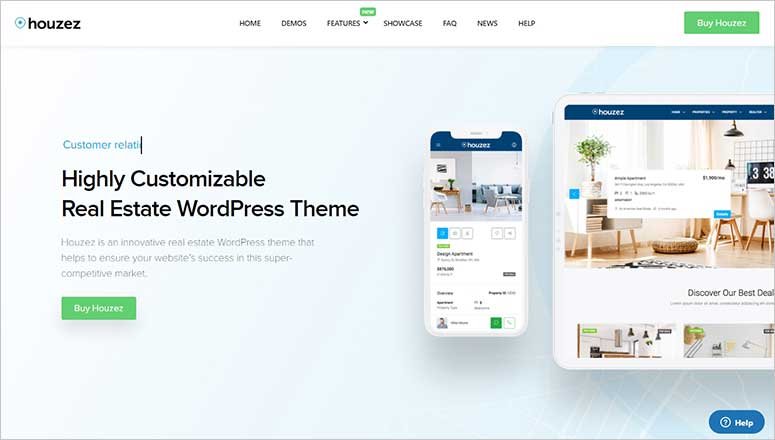The webpage titled 'Houses'—spelled H-O-U-Z-E-Z—features a distinct logo with a small blue accent next to it, situated at the top left corner. Centrally located at the top of the page are navigation tabs labeled Home, Demos, Features (with a new green icon above it), Showcase, FAQ, News, and Help. On the top right, a prominent green button labeled "Buy Houses" stands out.

Beneath these tabs, the main content highlights the theme's capabilities, stating "a highly customizable real estate WordPress theme." Despite some text being partially cut off, it further elaborates: "Houses is an innovative real estate WordPress theme that helps to ensure your website's success in this super competitive market." Another green button labeled "Buy Houses" is positioned below this description.

To the right of this central text, examples of customizable webpage themes are displayed. One theme is shown on a mobile phone and the other on a tablet, each presenting images of rooms furnished elegantly along with detailed listing information.